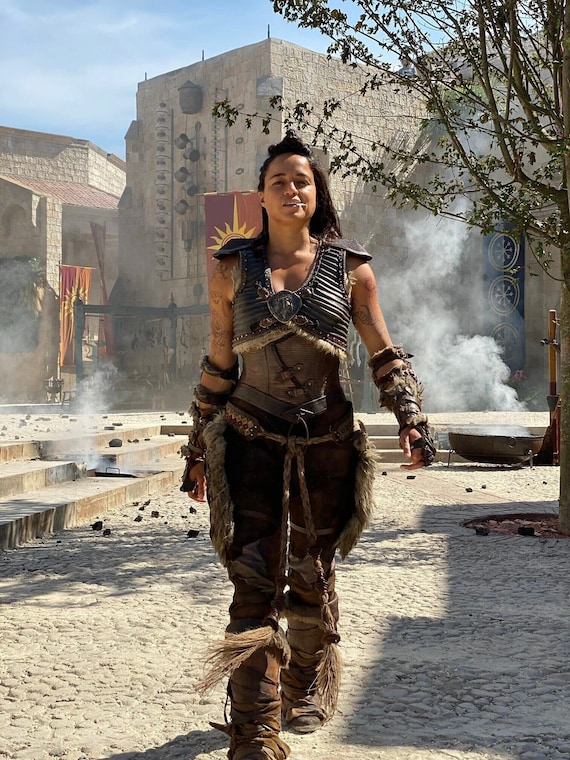The image showcases a woman dressed in what appears to be Viking-era inspired battle armor, walking towards the camera on a gray cobblestone street in a village setting. The woman has olive-toned skin, dark brown shoulder-length hair, partially pulled up with the rest cascading behind her. She is wearing a black vest with shoulder pads and an insignia, coupled with dark brown clothing on her torso and a combination of leather and metal armor adorned with fur. Her outfit includes black and brown belts, the latter holding an animal pelt at the back, leather pants, loose fabric boots, and dark brown arm guards extending from her hands up to her elbows. She appears to have a toothpick or similar object held in her mouth. Behind her, the village features stone buildings with steps leading up to them and red flags depicting a stylized yellow sun. Several columns of smoke rise from the buildings, adding to the rustic, medieval ambiance. The scene is bathed in sunlight with a clear blue sky dotted with fluffy white clouds, a tree partially extending into the upper right corner of the image. The setting suggests a large, open outdoor area devoid of other people, enhancing the focus on the solitary, armored woman.